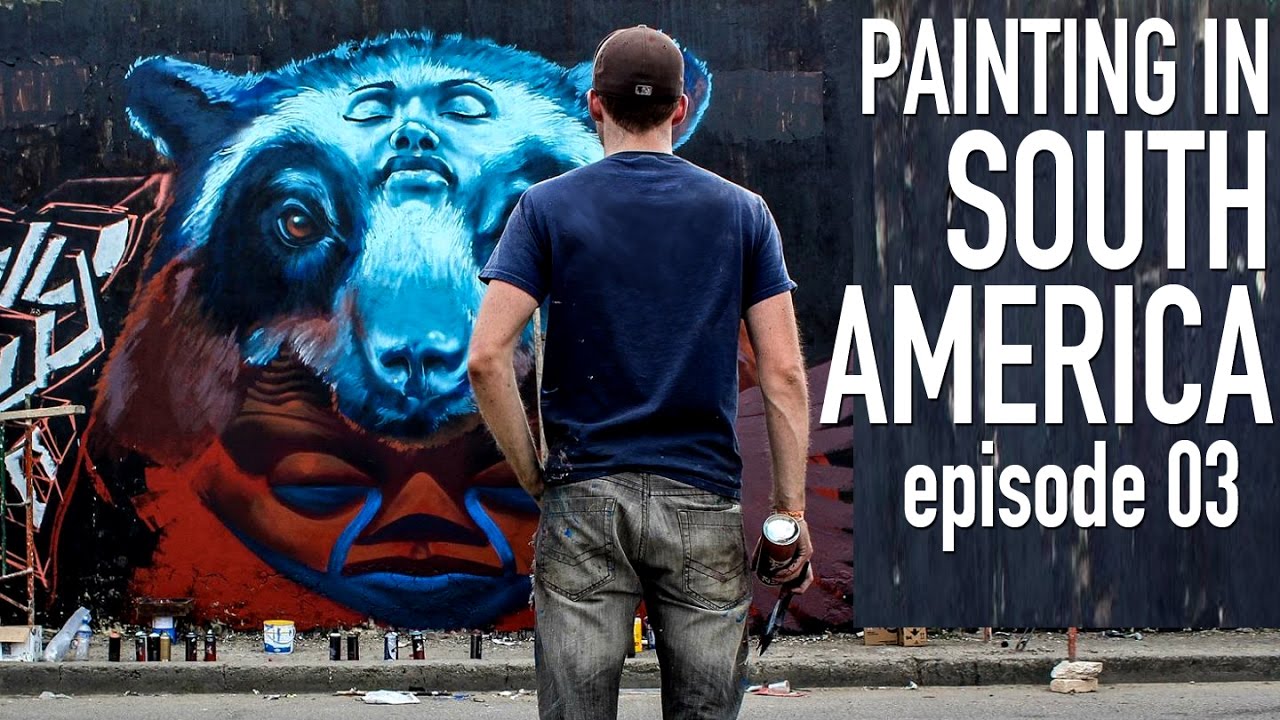In this urban scene, a man, dressed in a navy blue t-shirt, a brown baseball cap, and dirty gray jeans, stands in the street facing away from the camera. His left hand is in his pocket, while his right hand holds a can of spray paint, suggesting he is the artist behind the mural before him. The ground around him is strewn with approximately ten spray cans positioned along the edge of a curb, amidst scattered rocks, dirt, and debris, indicating a gritty street environment.

The mural on the wall displays a striking, hybrid image—a detailed blue bear with fur extending to rounded ears, featuring a human face with large closed eyes and prominent facial features embedded within its forehead. Beneath this, the image blends into another form, possibly a tribal face or a bare, meshed photograph, contributing to the mural's intricate design. Large, prominent white text on the right side of the mural reads, "Painting in South America, Episode 03," suggesting it might be part of a series or an advertisement for a TV show. This colorful and urban scene vividly showcases the artistry and raw creativity of urban graffiti culture.